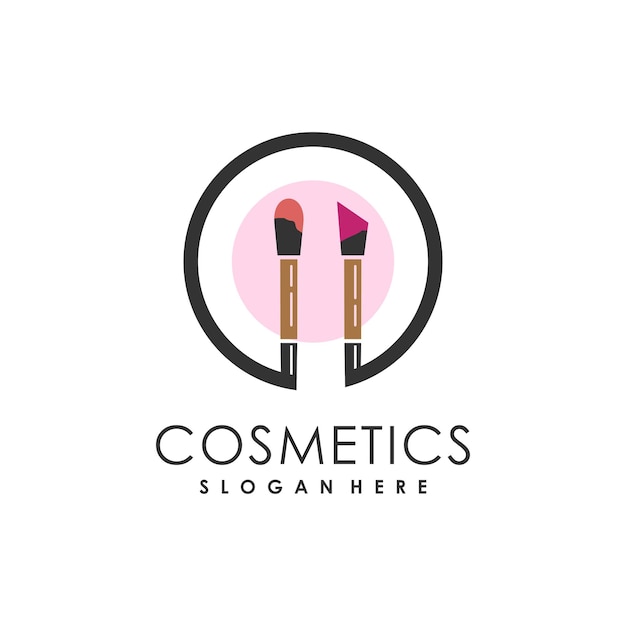The image is a highly minimalistic yet effective advertisement for cosmetics, set against a white background. The central focus is a black circle housing a pink center with a white ring encircling the pink. Positioned vertically side by side, two different types of cosmetic brushes connect to the black circle. One is an angled flat brush tipped with a lavender or dark pink cosmetic, while the other is a rounded brush whose tip holds a brownish colored cosmetic, both appearing almost in a cartoon fashion. Below the image, in bold black lettering, is the text "Cosmetics," followed by the line "Slogan Here." The entire composition exudes simplicity and elegance, emphasizing the brand's modern aesthetic.